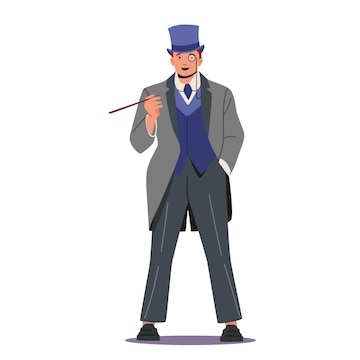The image depicts a detailed, animated sketch of a fashionable gentleman centered against a white background. The man, whose skin is white and hair appears brown, is adorned in a gray suit comprising a gray suit coat and gray slacks. His attire is complemented with a blue shirt and tie. He stands confidently, his left hand tucked into a pocket while his right hand holds an elegant cigarette holder. A monocle is delicately perched on his left eye, attached to his suit jacket. Completing his sophisticated look, he wears a purple top hat snugly on his head and a matching purple vest. His ensemble is rounded off with black dress shoes as he stands on a subtle blue platform. The sketch artist has skillfully highlighted his distinguished appearance, blending elements of classic gentlemanly attire with a touch of whimsical charm.